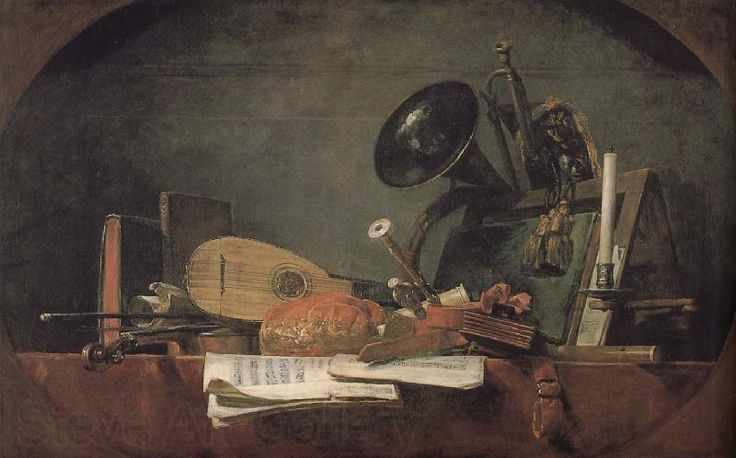The painting presents an arrangement of various musical instruments meticulously placed atop a wooden table, bathed in a naturalistic and somewhat somber palette of browns, whites, blacks, oranges, silvers, golds, grays, tans, and greens. Dominating the scene is a wooden acoustic guitar complemented by a large brass horn resting centrally. There is also a flute, identifiable by its sleek and slender design. Scattered across the table are several brown books, one of which has sheets of musical notation cascading off the edge, providing hints of the melodies they contain. A candle, unlit yet evoking a sense of tranquility, stands beside these books. A violin's bow lays nearby, enhancing the musical theme. Additionally, a belt dangles off the table's side, adding a touch of casual realism. At the table's back, what might be an easel or music stand holds its ground. The background is a muted greenish-gray, allowing the objects in the foreground to stand out vividly. This piece, likely oil-based, is not excessively bright but uses its darker, more natural hues to achieve a sophisticated and serene ambiance, suitable for a gallery or a refined household setting.